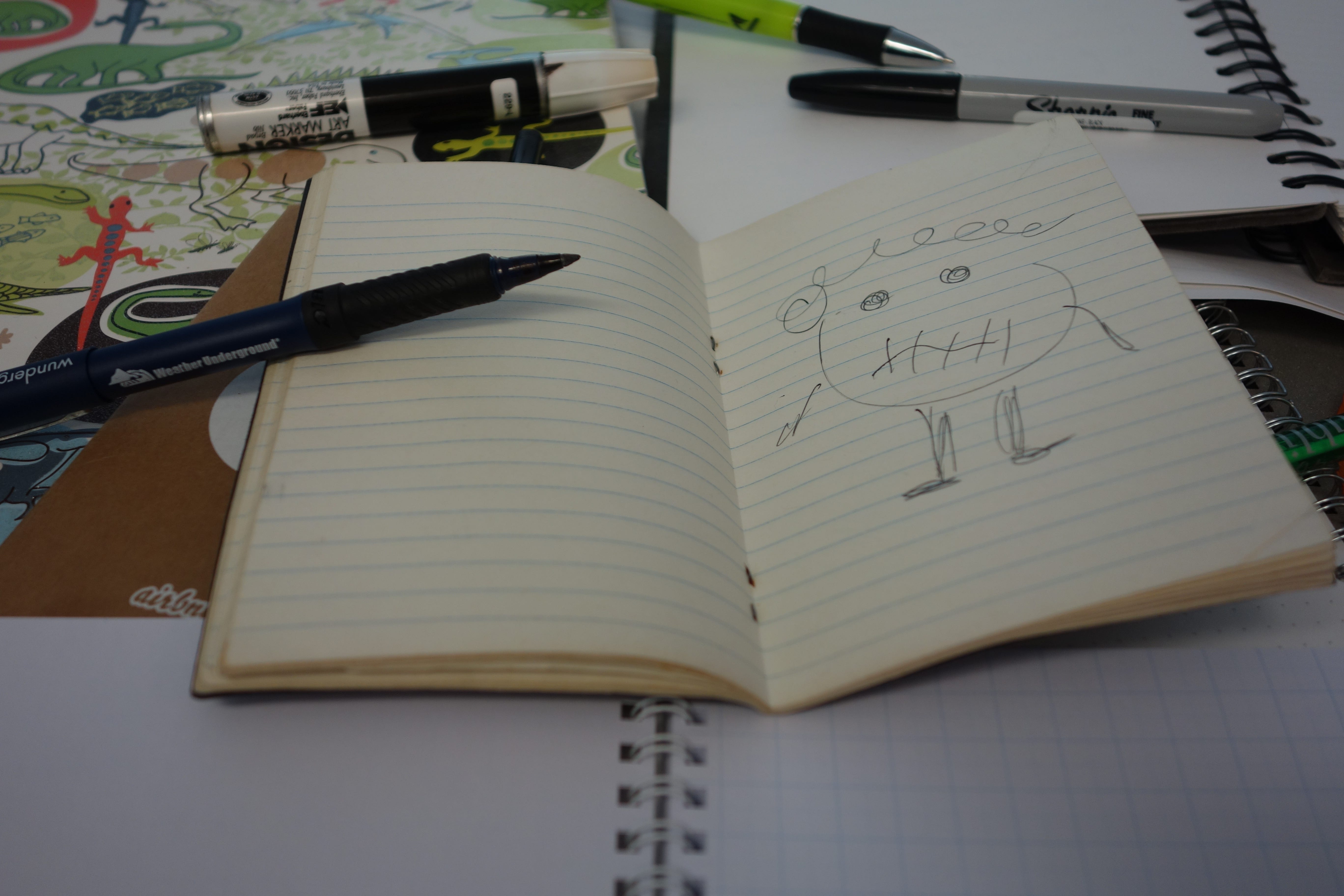The photograph features an opened journal booklet, prominently displayed in the center. Leaning against one of the pages are a black and a blue pen. The focus of the journal page is a cartoon sketch of a small, round character with squiggly hair, round dark eyes, and a stitched-shut mouth. The character has short, stubby legs and arms that extend out from either side of its body.

In the background, there is an assortment of pens, including a Sharpie, another pen, and what appears to be an art marker. Several open workbooks and sketchbooks are layered underneath the journal, giving the scene a creative and busy atmosphere. To one side of the setup, a very colorful surface or book cover is visible, adorned with cartoon illustrations of various animals, lizards, and dinosaurs on a white background, adding a lively and whimsical touch to the composition.